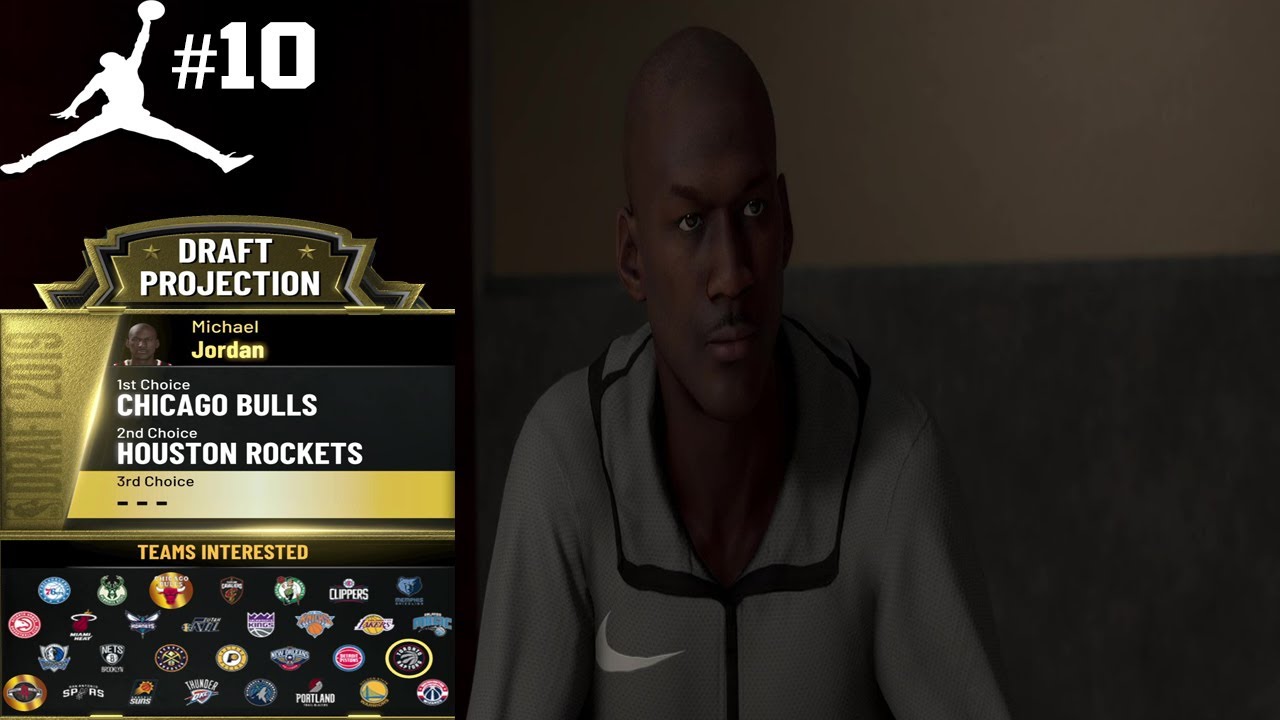This image is a screenshot from a video game, featuring a detailed draft projection for legendary basketball player Michael Jordan. At the top left corner of the screen, the number "10" is prominently displayed. Below that, there is a silhouette of Michael Jordan mid-leap, extending his hand towards a basketball hoop, effectively capturing him in the iconic act of shooting a basketball.

Adjacent to the silhouette, text reads "Draft Projection," with "Michael Jordan" written underneath. Down the left side of the screen, the draft details outline the 2019 draft prospects: Jordan is highlighted as the first choice for the Chicago Bulls and the second choice for the Houston Rockets. The third choice remains unspecified, represented by three dashes.

Towards the bottom, a list of team emblems showcases the various teams interested in Jordan. The emblems are arranged in four rows: the first and third rows contain seven team logos each, while the second and fourth rows include eight logos each.

On the right side of the screen, there is a digitally-rendered image of Michael Jordan wearing a Nike swoosh shirt, providing a modernized visual representation of the basketball legend.